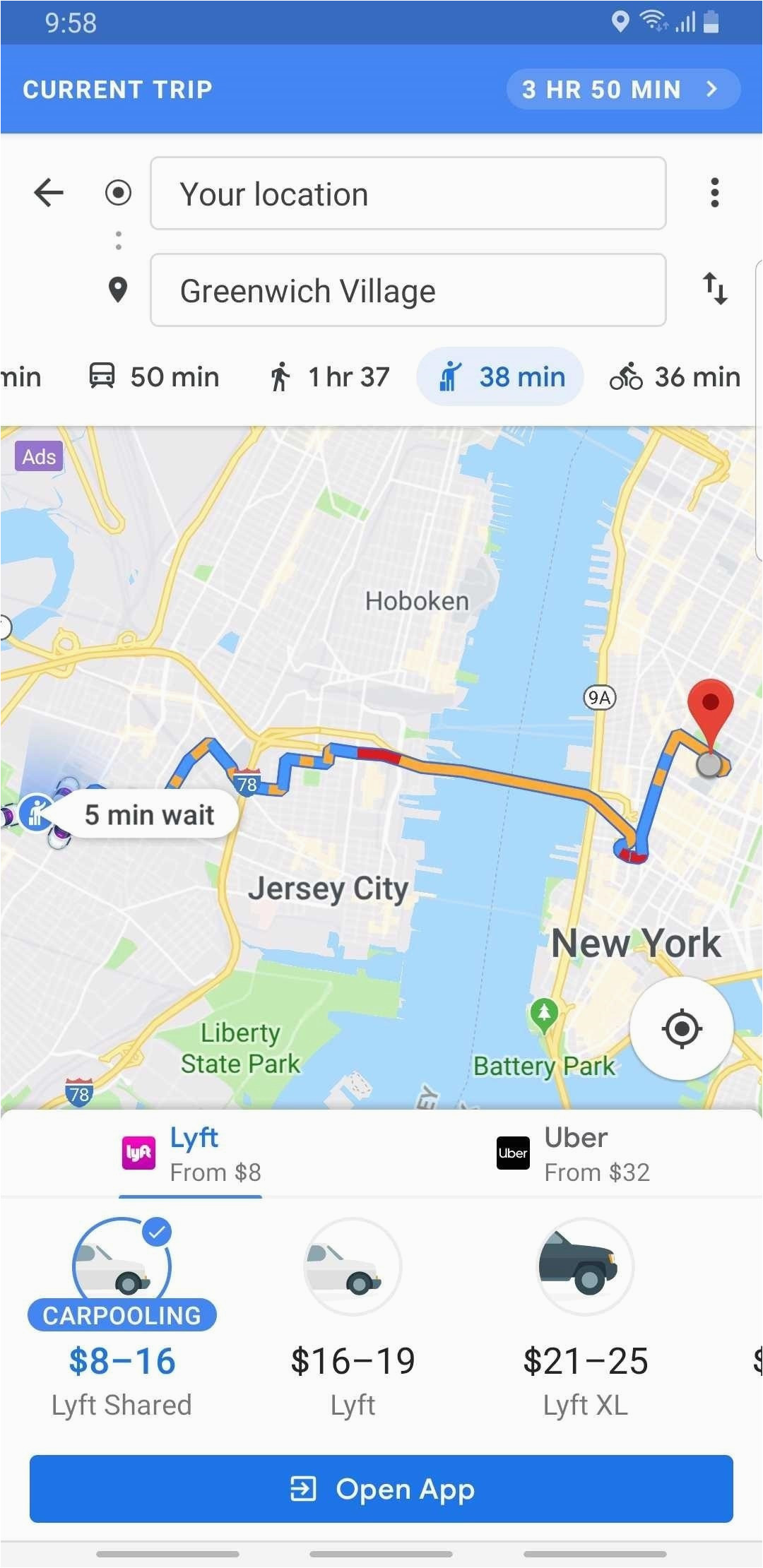The image displays a phone screen with detailed Lyft pricing information for vehicle transportation. At the top left, the price is listed as $9.58. The top right corner shows icons for wireless signal, cellular signal, and battery strength, with the battery more than halfway depleted. 

The screen indicates a current trip duration of 3 hours and 50 minutes. A text box labeled "Your location" is shown, followed by another box indicating "Greenwich Village." Below, a time estimate of 38 minutes is highlighted.

A map is displayed, with Jersey City on the left side and New York City on the right. The map outlines a route starting in New York and crossing a body of water to Jersey City. On the far left, it mentions a 5-minute wait time.

Pricing options are listed below:
- A highlighted option for "Lyft" with the logo, starting from $8.00.
- On the right, "Uber" pricing begins from $32.00.
- A circle icon with a car and a check mark, labeled "Carpooling, $8-$16.00 Lyft Shared."
- Another circle with a car, indicating "Lyft $16-$19.00."
- A circle with a black vehicle, labeled "Lyft XL $21-$25.00."

At the bottom of the screen, a blue rectangle displays the text "Open App."